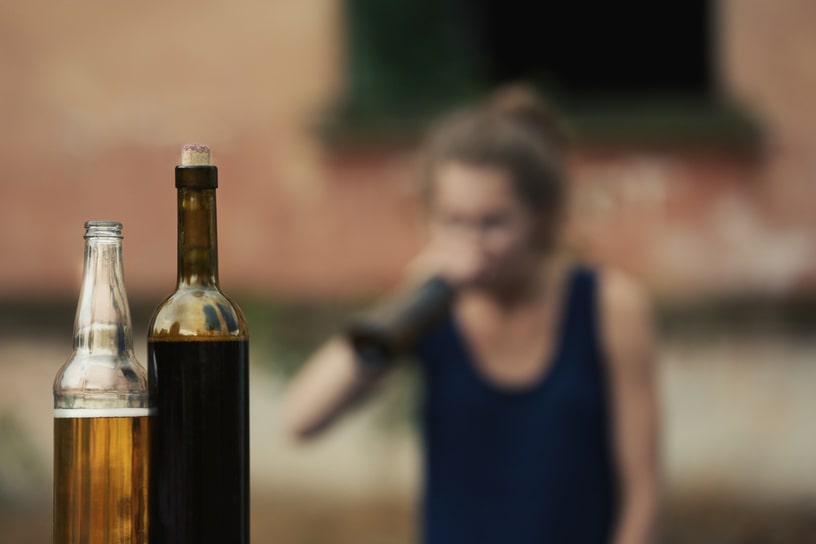This close-up photograph captures a compelling scene with a woman in the blurry background and two distinct bottles of alcohol in the sharp foreground. The woman, who appears to have her hair pulled up and is wearing a black tank top, is drinking from a bottle held horizontally to her lips, suggesting she has just started drinking. Her blurred figure, set against a worn brick building with peeling paint and a green trim, emphasizes the focus on the bottles in front. 

The bottle to the left is a clear container filled halfway with a light amber liquid, possibly beer, and it has an open screw cap. The taller bottle on the right, which contains a very dark liquid reminiscent of deep blue or almost black wine, remains sealed with a cork. The setting appears to be outdoors, enhancing the photograph's candid and spontaneous nature.